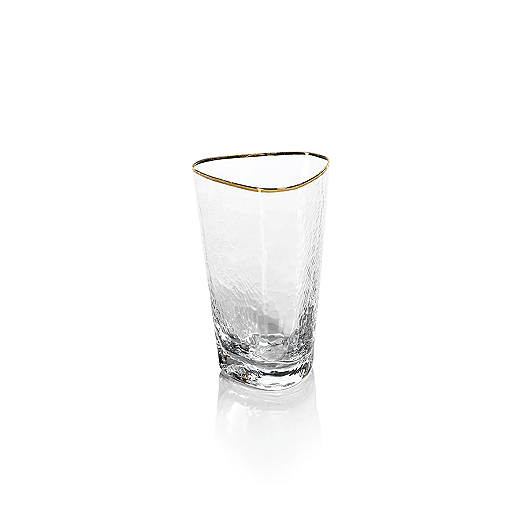This image features a clear, triangular-shaped glass set against a stark white background. The glass is adorned with a thin gold rim at its irregularly shaped lip, adding a hint of elegance. The glass itself has a fascinating pattern that mimics the appearance of shattered glass or scales, though it remains intact. At the bottom of the glass, small, partially melted ice cubes or liquid are visible, enhancing the overall texture. The surface beneath the glass is somewhat reflective, casting a faint reflection of the glass. The minimalist setting with no visible light source emphasizes the intricate details and unusual design of the glass.